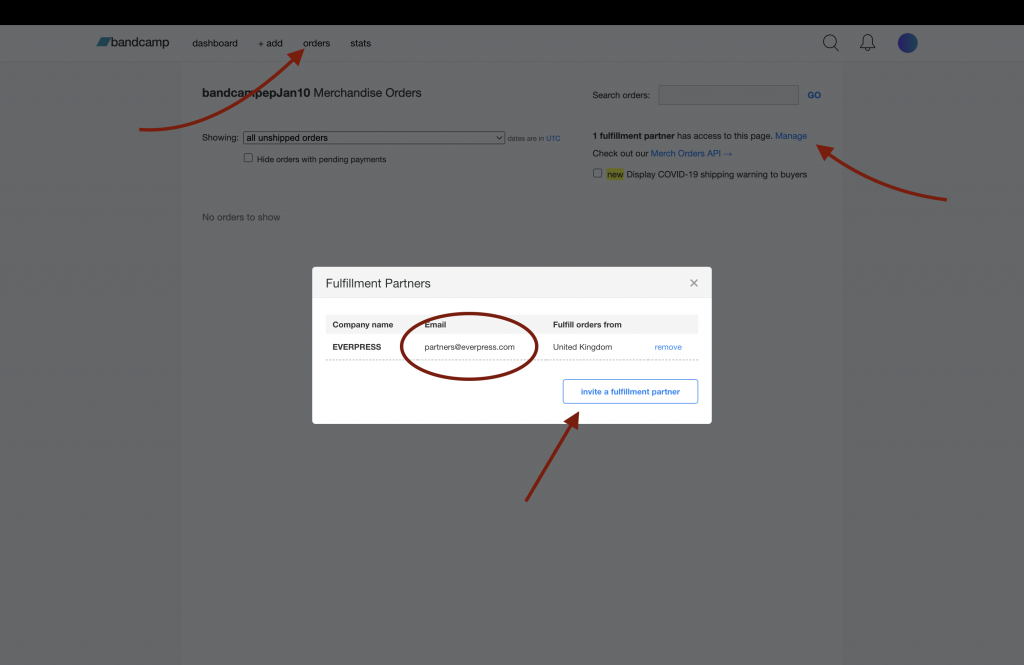The image captures a web page overlaid with a pop-up message, which grays out the background making it difficult to view. The web page in the background appears to be the "Bandcamp Dashboard," discernible from the header at the top. An item on the page is highlighted with a red arrow, although its specifics are unclear. In the upper right corner of the page, there are icons of a magnifying glass, a notification bell, and a round blue profile picture. Below these icons is a text box followed by a sentence, also marked by a red arrow. 

The pop-up, which has a rectangular shape, reads "Fulfillment Partner" and contains several text elements. It mentions the company name "EverPress" alongside an email address that is too small to read but is circled. It also includes the phrase "Fulfill Orders" and notes "United Kingdom." At the bottom right of the pop-up, there is a box labeled "Invite a Fulfillment Partner," which is indicated by another red arrow.